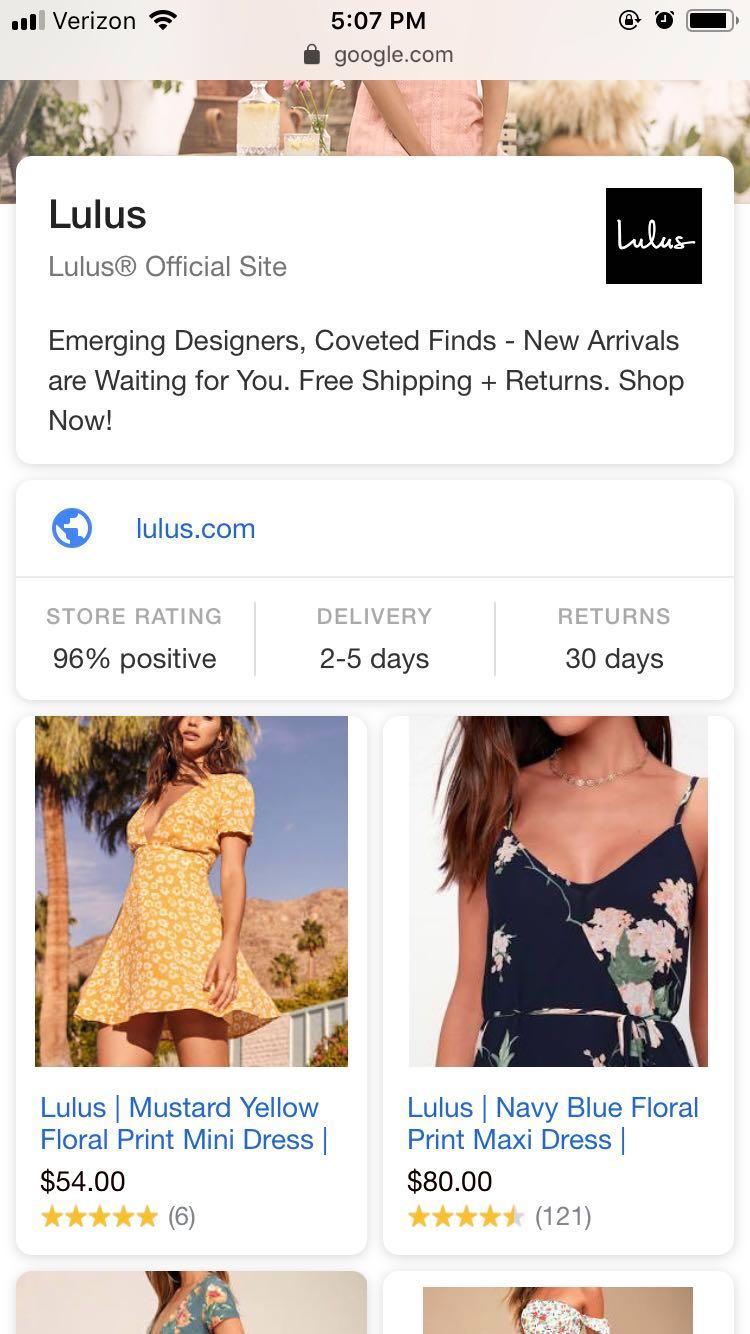A smartphone screenshot displays a website, clearly identifiable as such due to the 'Verizon' carrier indicator on the top left, a time reading of 5:07 PM in the middle, and a nearly fully charged battery at approximately 92% on the top right. The webpage shown belongs to a store named Lulu's, with the URL Lulu's.com. At the top left of the webpage, it reads "Lulu's - Our Official Website," followed by marketing text promising "Emerging designers, coveted finds, no rivals are waiting for you. Free shipping plus returns. Shop now."

The top right of the webpage features Lulu's logo, a black square with the name "Lulu's" written in cursive. Below this logo is a link to Lulu's.com, presumably the same site currently being viewed. Towards the bottom of the screenshot, there is a section with customer ratings and store policies: a store rating of 96% positive, delivery times of 2 to 5 days, and a 30-day return policy.

Additionally, two product listings are visible at the bottom of the page. On the left is a "Lulu's Mustard Yellow Floral Print Mini Dress," priced at $54. To the right is a "Lulu's Navy Blue Floral Print Maxi Dress," priced at $80.